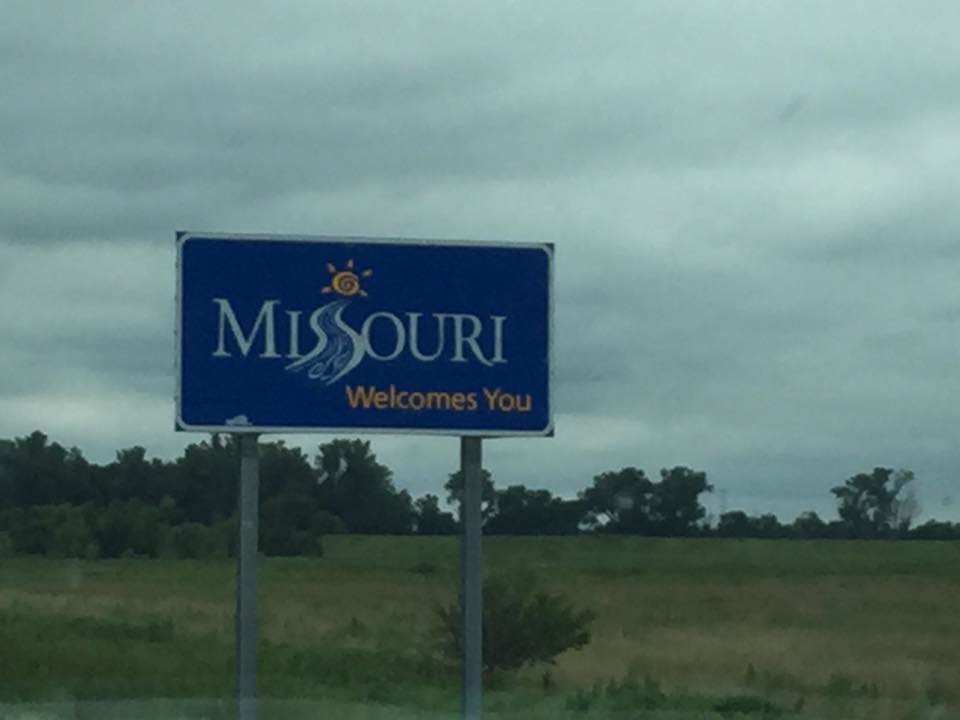This photograph captures a vivid outdoor scene featuring a prominent road sign situated on a patch of green grass, interspersed with some shrubs. In the distance, a backdrop of trees is visible. The sky overhead is entirely overcast, shrouded in gray clouds. Positioned on the left side of the image, the sign is supported by gray posts. The sign itself is predominantly blue and centrally displays the word "Missouri," with the 'S' in Missouri creatively stylized to resemble a flowing river. Above this artistic 'S,' there is a graphic depicting a sun. Below the word "Missouri," the phrase "welcomes you" is neatly inscribed, slightly offset towards the right side of the sign.